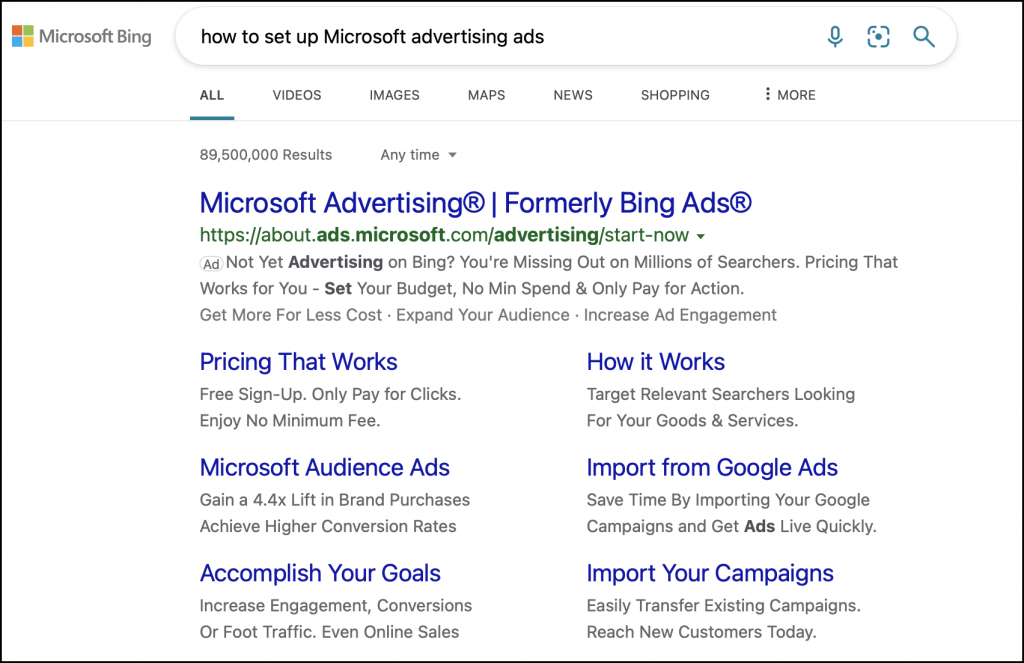The image is a screenshot of a Microsoft Bing search engine page. Prominently displayed is the Microsoft logo, featuring the iconic red, green, blue, and yellow squares. The search bar contains the query "how to set up Microsoft Advertising ads," and next to it are blue icons for a microphone (voice search), a camera (image search), and a magnifying glass (search). At the top, there are tabs labeled "All," "Videos," "Images," "Maps," "News," "Shopping," and "More," with "All" underlined in blue. The "More" tab is accompanied by three dots. The search has yielded approximately 89,500,000 results. Also visible is an "Anytime" drop-down button. A prominent advertisement for Microsoft Advertising, formerly Bing Ads, appears at the top of the search results. It includes a green hyperlink and informational phrases such as "Pricing that Works," "Microsoft Audience Ads," "Accomplish Your Goals," "How It Works," "Import from Google Ads," and "Import Your Campaigns."